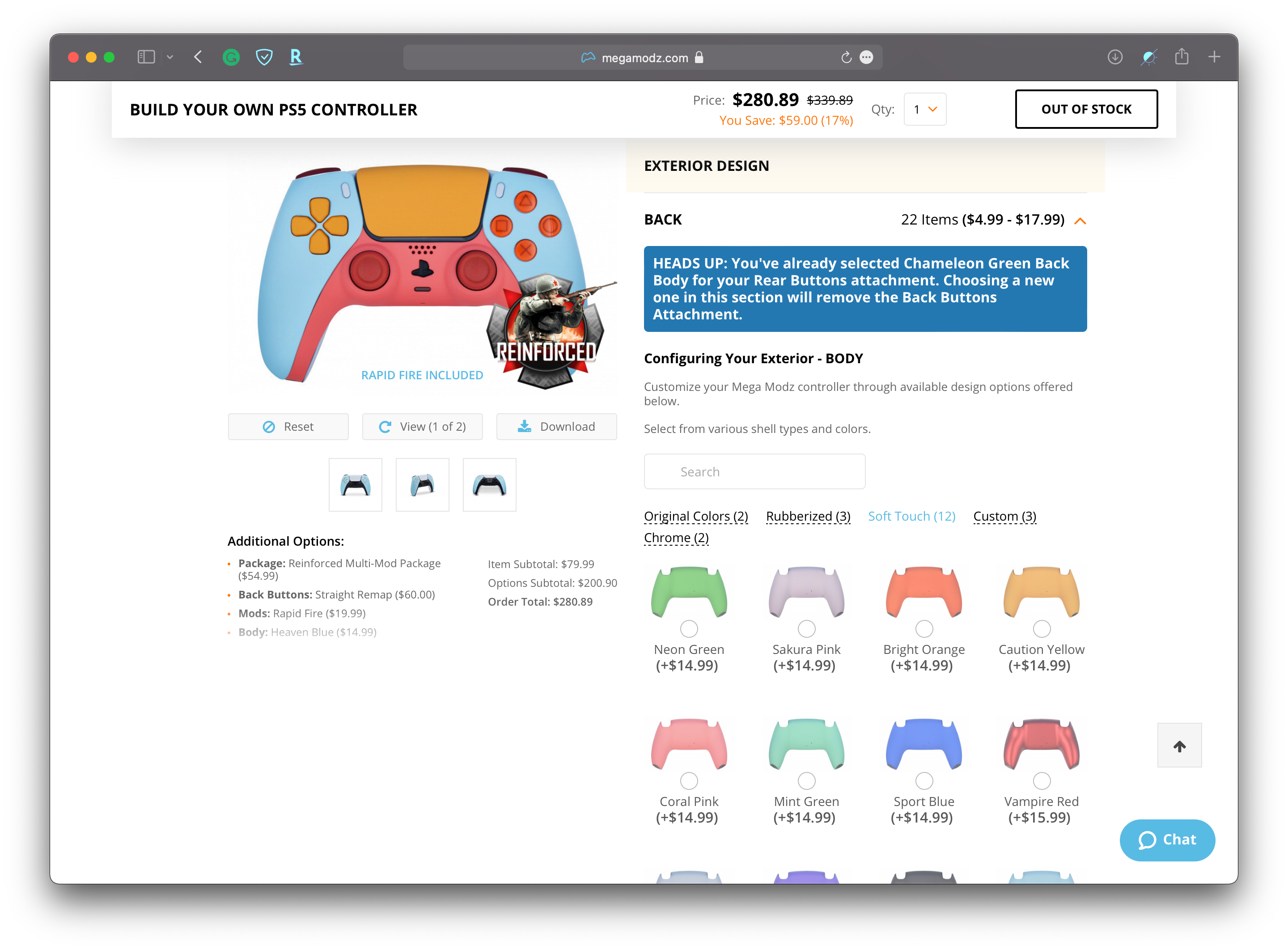The image showcases a website titled "Mega Mods" at the top bar, which is displayed in a Mac interface, identifiable by the distinct red, yellow, and green buttons located in the top-left corner of the window. Below the address bar, the main webpage focuses on custom video game controllers, particularly highlighting a PlayStation 5 controller on the top left corner.

The section prominently displays an option to "Build Your Own PS5 Controller," with pricing details indicating a discounted price of $288, down from the original $339.89. The discount is marked in yellow, showing a savings of $59, which is equivalent to 17%. There is a note stating that the quantity available is currently out of stock. 

The featured PS5 controller has a vibrant and unique design: the center is orange, the bottom area is red, and the handle areas on both sides are blue, adorned with yellow and orange buttons. A small image of a soldier reinforces the customized appearance, suggesting a robust and fortified design. Additional thumbnail images display various angles of the controller, offering more visual perspectives.

On the right side of the page, there are customization options under "Exterior Design" and "Back." A notification warns that the selection of a new back design will remove the chameleon green back body already chosen for the rear buttons attachment. Below this, various back attachment options and their respective prices are listed for further customization.